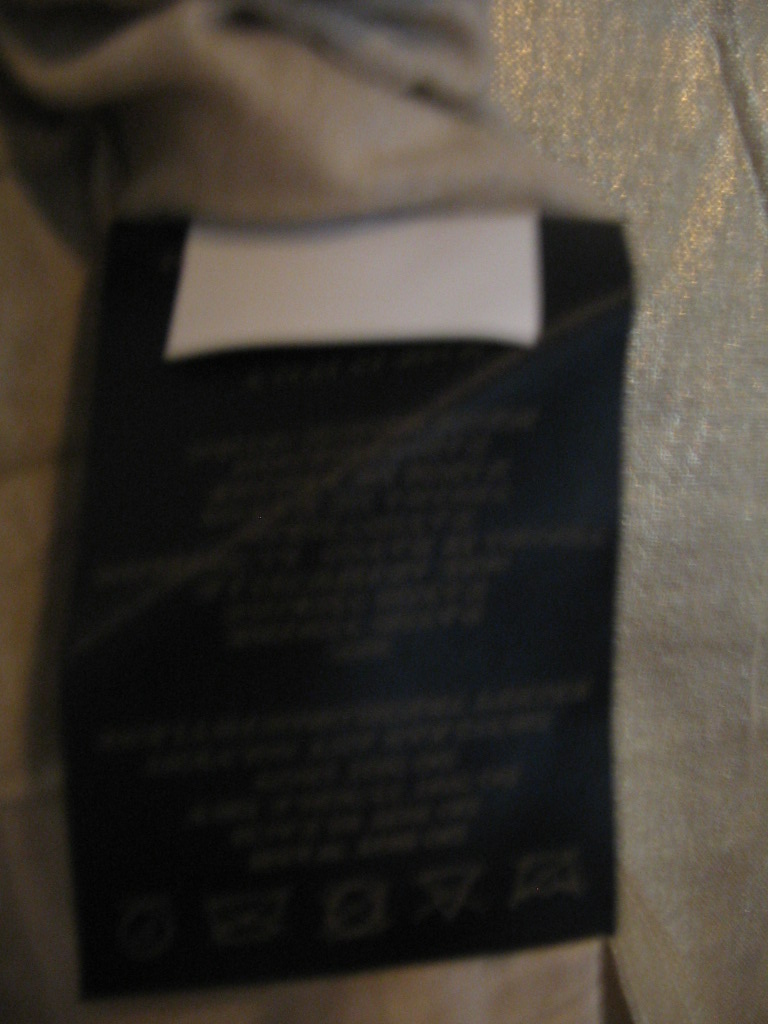This photo is extremely blurry, making it difficult to discern specific details. It depicts a close-up of what appears to be a black clothing care tag with gold lettering and various symbols that likely provide instructions on how to care for the garment. Directly above this black tag, there is a small white tag whose contents are indiscernible but might be a size tag. The garment to which these tags are attached seems to be a very light tan or pale mauve color with hints of gold. The overall appearance suggests that this is a zoomed-in shot of a clothing tag, yet due to the poor image quality, the precise details are hard to define.